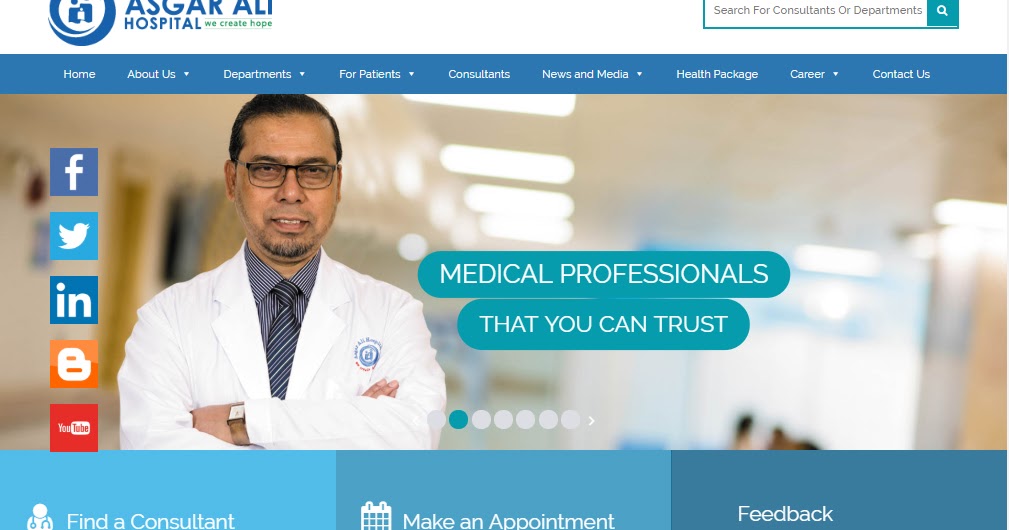Homepage of Asghar Ali Hospital's Website

The homepage of Asghar Ali Hospital's website features a visually appealing layout dominated by shades of blue, conveying a sense of trust and tranquility. Central to the page is a stock photo of a Middle Eastern male doctor, characterized by a thin beard, glasses, and a professional demeanor in a white lab coat. The tagline "We create hope" is prominently displayed, reinforcing the hospital's commitment to patient care.

Adjacent to the doctor's image is a bold statement: "Medical professionals that you can trust," emphasizing the credibility and expertise offered by the hospital's staff. At the bottom of the image, there are three interactive buttons designed for user convenience: "Find a Consultant," "Make an Appointment," and "Feedback."

The top-right corner of the page hosts a search bar, facilitating easy navigation. Directly below it, a comprehensive menu includes the following subsections: About Us, Departments, For Patients, Consultants, News & Media, Health Package, Career, and Contact Us. These sections provide detailed information and resources for both current and prospective patients.

On the left side of the page, beside the doctor's image, is a cluster of social media icons, directing visitors to Asghar Ali Hospital's Facebook, Twitter, LinkedIn, YouTube, and Blogger profiles. This integration enables users to stay updated and connected through their preferred social media platforms.

Overall, the website's design is clean, user-friendly, and exudes professionalism, making it easy for visitors to find the information they need and take necessary actions.